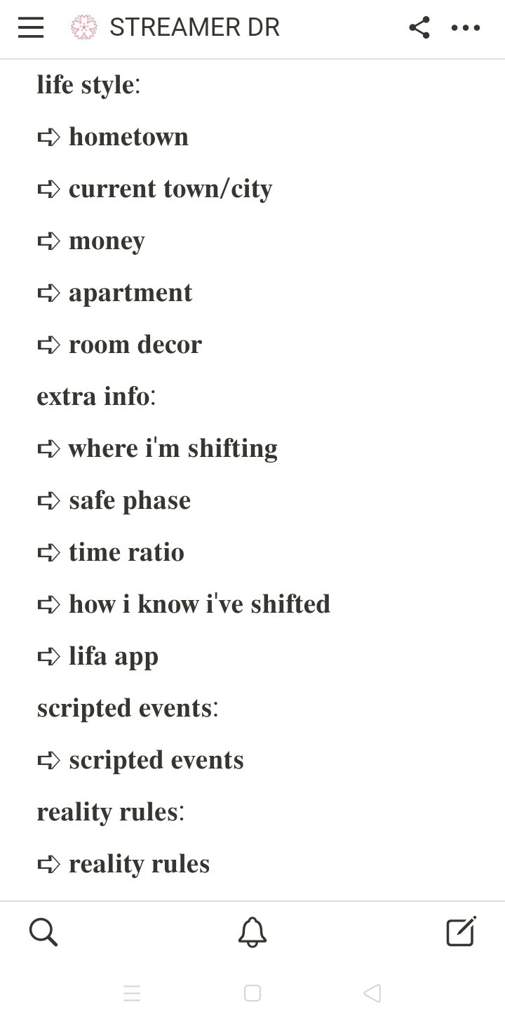This is a detailed screenshot of a mobile application interface related to a streamer named "DR". At the top of the screenshot, there is a hamburger menu icon beside the name "STREAMER DR" in all capitals. Adjacent to the name are a share button and a three-dot options button. The text is basic black on a white background. The header "lifestyle:" appears, followed by several categories presented with arrow bullet points. The categories include: hometown, current town city, money, apartment, room decor. 

Further down, there is another section titled "extra info" which includes additional bullet points for: where I'm shifting, safe phase, time ratio, how I know I've shifted, and Leafa app. Another category labeled "scripted events" has one arrow bullet point titled "scripted events". Similarly, "reality rules" has a single bullet point titled "reality rules".

At the bottom of the screen, there are three icons: a search icon, a bell for notifications, and an edit button.